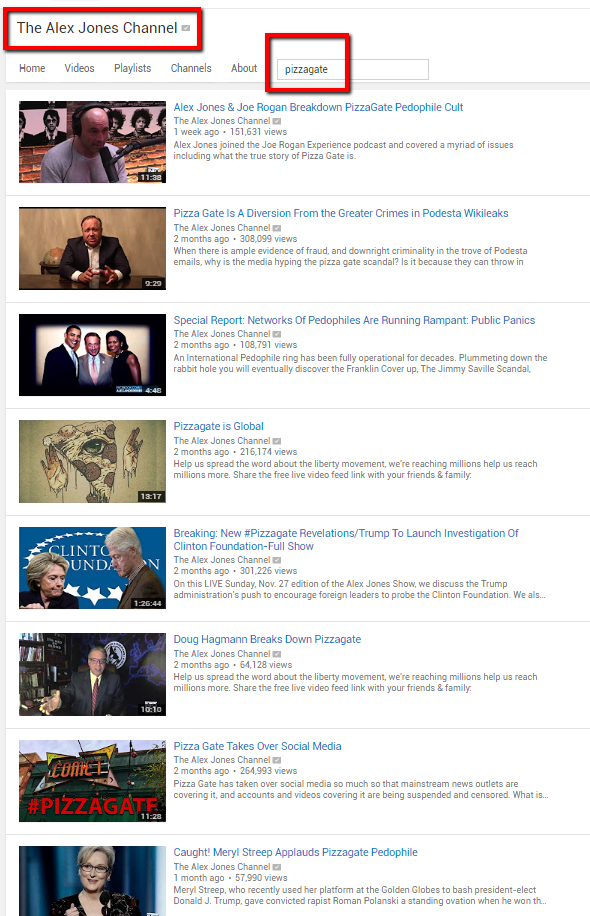At the top of the image, a long rectangle outlined in red displays "The Alex Jones Channel." Beneath this heading, a horizontal menu bar includes options such as Home, Videos, Playlists, Channels, and About. Adjacent to these options, there is a search bar with the term "Pizzagate" typed inside, also encased in a red square.

Below the menu bar, various video thumbnails are shown. The first video is titled "Alex Jones and Joe Rogan Break Down Pizzagate Pedophile," featuring an image of Joe Rogan seated with a microphone in front of him, presumably for a podcast. 

The subsequent video category includes a title, "Pizzagate is a Diversion from the Greater Crimes in Podesta WikiLeaks," followed by another titled "Special Report: Networks of Pedophiles Are Running Rampant."

Next, the video titled "Pizzagate and Global," includes an image of Hillary and Bill Clinton. Following this, another video is titled "Breaking: New Pizzagate Revelations."

Underneath these, another video titled "Doug Hagmann Breaks Down Pizzagate" is shown, followed by "Pizzagate Takes Over Social Media, #Pizzagate."

Finally, the last video thumbnail is titled "Caught: Meryl Streep Pizzagate Pedophile," featuring her image beside the title.